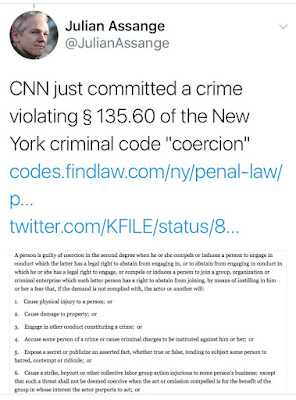**Caption:**

In this image, Julian Assange, the founder of WikiLeaks, is depicted at an event. Recently, CNN has been accused of violating Section 135.60 of the New York Penal Law, which addresses coercion in the second degree. According to the code, a person is guilty of coercion when they compel or induce someone to engage in or abstain from engaging in conduct to which they have a legal right. This can involve threats to commit a crime, accusations of a crime, exposure of secrets, or causing strikes or boycotts. The violation implies exerting improper pressure on an individual to influence their actions against their legal rights.